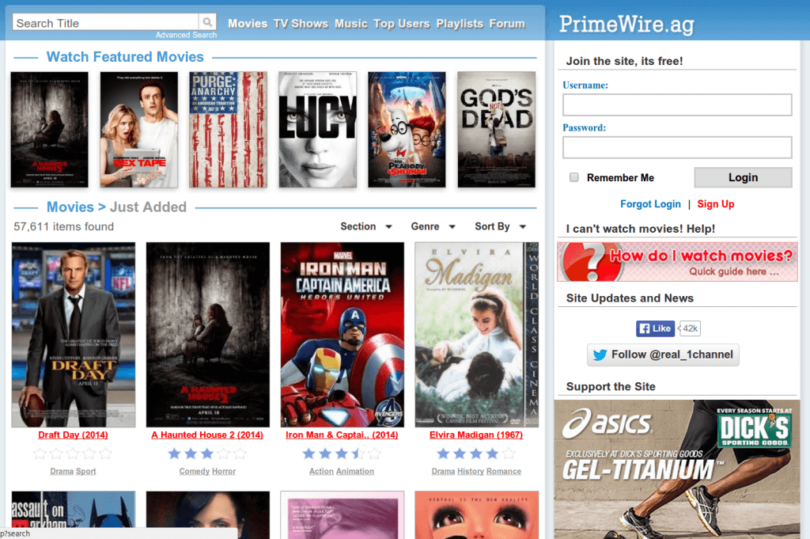The image appears to be a screenshot of a website, likely named "primewire.at," which seems dedicated to streaming video content such as movies and TV shows. The top section features a blue banner that spans the width of the page. Positioned at the upper right corner of this banner, there is a white search box accompanied by a button with a magnifying glass icon.

Directly beneath the banner, a navigation menu in white text offers links to various sections: Movies, TV Shows, Music, Top Users, Playlist, Forum, and ends with the primewire.at logo on the far right. Beneath the navigation menu, occupying about two-thirds of the left side of the screen, is the "Watch Featured Movies" section. This section displays a row of thumbnails, each representing different movies available for selection.

Below this section is another labeled "Movies Just Added," demarcated by a blue line. It showcases four movie thumbnails with titles partially visible, including "Craft Day," "Iron Man," "Captain America," and "Madigan." Each movie entry features a promotional image.

On the right side of the screen, taking up roughly one-third of the layout, there is a user login section positioned below the primewire.at branding. This section includes fields for username and password, a "Remember Me" checkbox, and a "Login" button. Additionally, there are links for "Forgot Login?" in blue text and "Sign Up" in red text.

Further down, there is a "I can't watch movies, help" section, followed by information related to Facebook, and an invitation to support the site through advertisements from VIX.